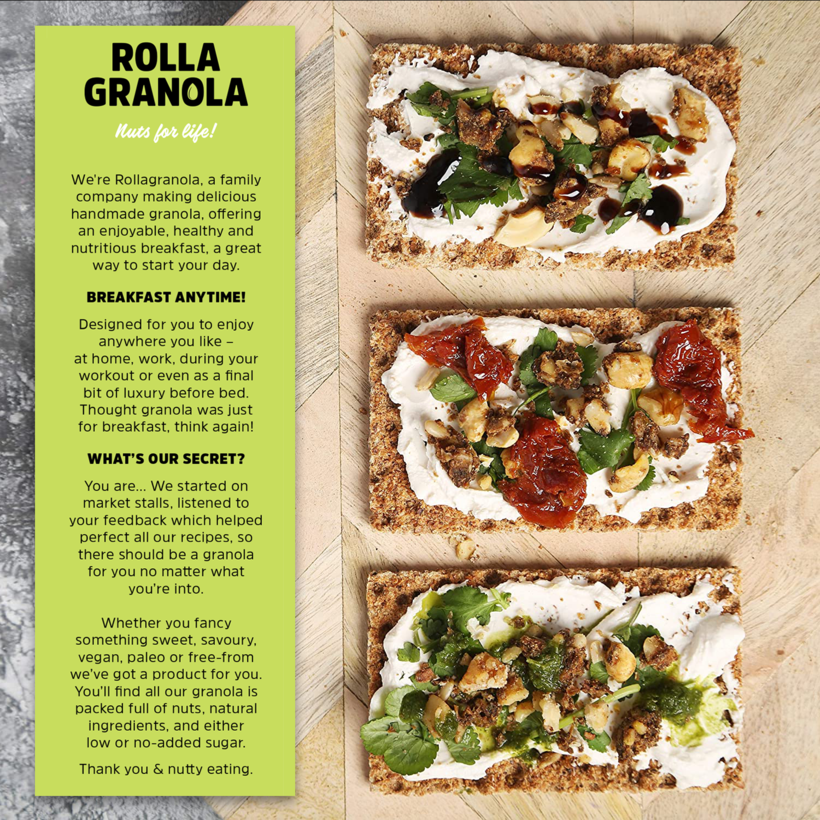The image features a detailed presentation of Rola Granola's products and company ethos, seemingly from a cooking or health magazine. The background is a light wooden surface that resembles a flat serving tray or cutting board. On the right-hand side, there are three vertically-stacked granola bars, each topped with a distinct combination of ingredients. The top bar has a white spread garnished with what appears to be black olives and a brown dressing. The middle bar has the same white spread, but is adorned with orange tomatoes, cranberries, and green herbs. The bottom bar features a simpler arrangement with the white spread, plain nuts, and herb leaves. Each bar aligns neatly, creating an appealing visual.

On the left-hand side, a rectangular, olive-colored section showcases Rola Granola's branding and philosophy. At the top, the text "Rola Granola, Nuts for Life" is prominently displayed in black. Below it, a detailed article describes the family-owned company’s dedication to creating delicious, handmade granola aimed at providing a healthy and nutritious breakfast option. The text emphasizes the versatility of their granola, suitable for any time of day, whether at home, during a workout, or as a nighttime snack. The company prides itself on listening to customer feedback to perfect their recipes, offering a range to cater to different tastes and dietary needs, including sweet, savory, vegan, paleo, and low or no added sugar options. The granola is highlighted for being packed full of nuts and natural ingredients.